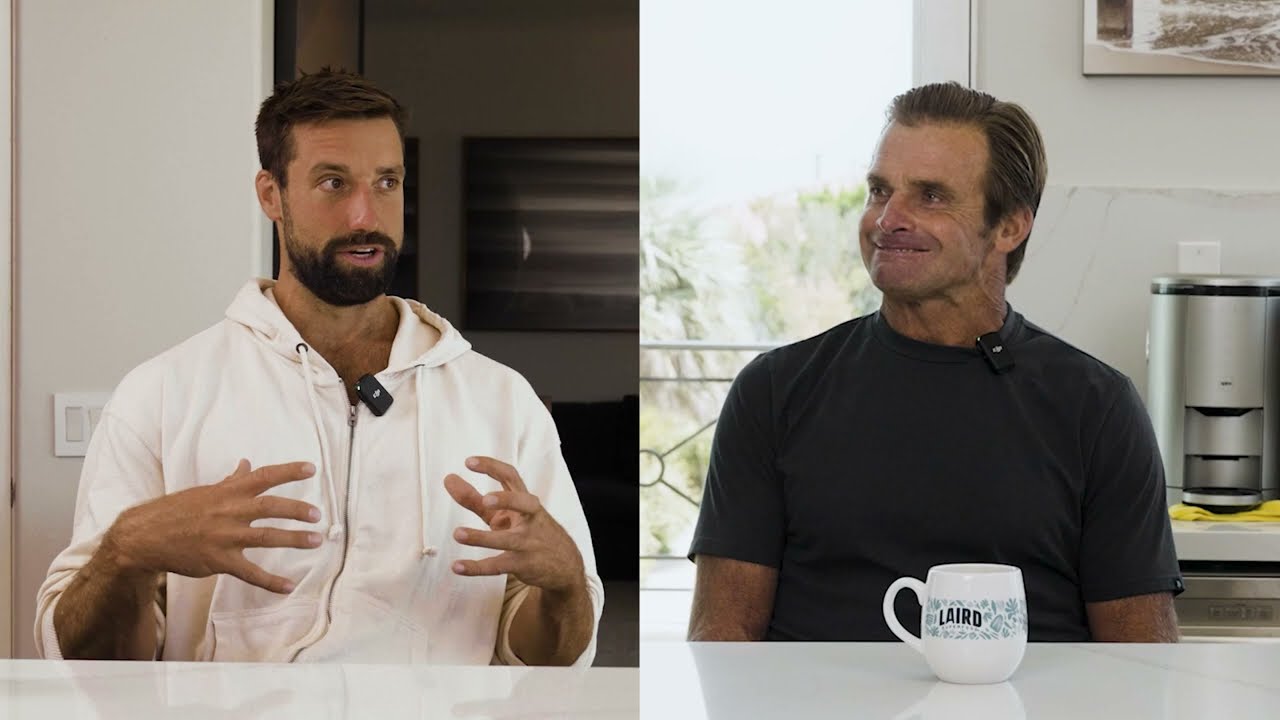This image shows a split-screen of a videoconferenced conversation between two men in separate locations, both with microphones clipped to their collars. The man on the left, who appears to be around his 40s, is wearing a white button-down shirt and gesturing with his hands in front of him. He has dark hair, a close-cut dark beard, and mustache. He is seated at a white table positioned in front of a white wall with a light switch. A black sofa and a portrait hanging on the wall are visible in the background. 

The man on the right, slightly older in his late 40s, is clean-shaven with brown hair. He is wearing a black t-shirt and sits at a white table or countertop with a white coffee mug in front of him that says "L-A-I-R-D." Behind him to the right is a silver coffee maker, and to the left is a glass door that leads to a balcony. Both men look different directions, and the man on the right seems to be grimacing or displaying a closed-mouth smile. The scene has all the visual cues of a virtual meeting or an online conversation.